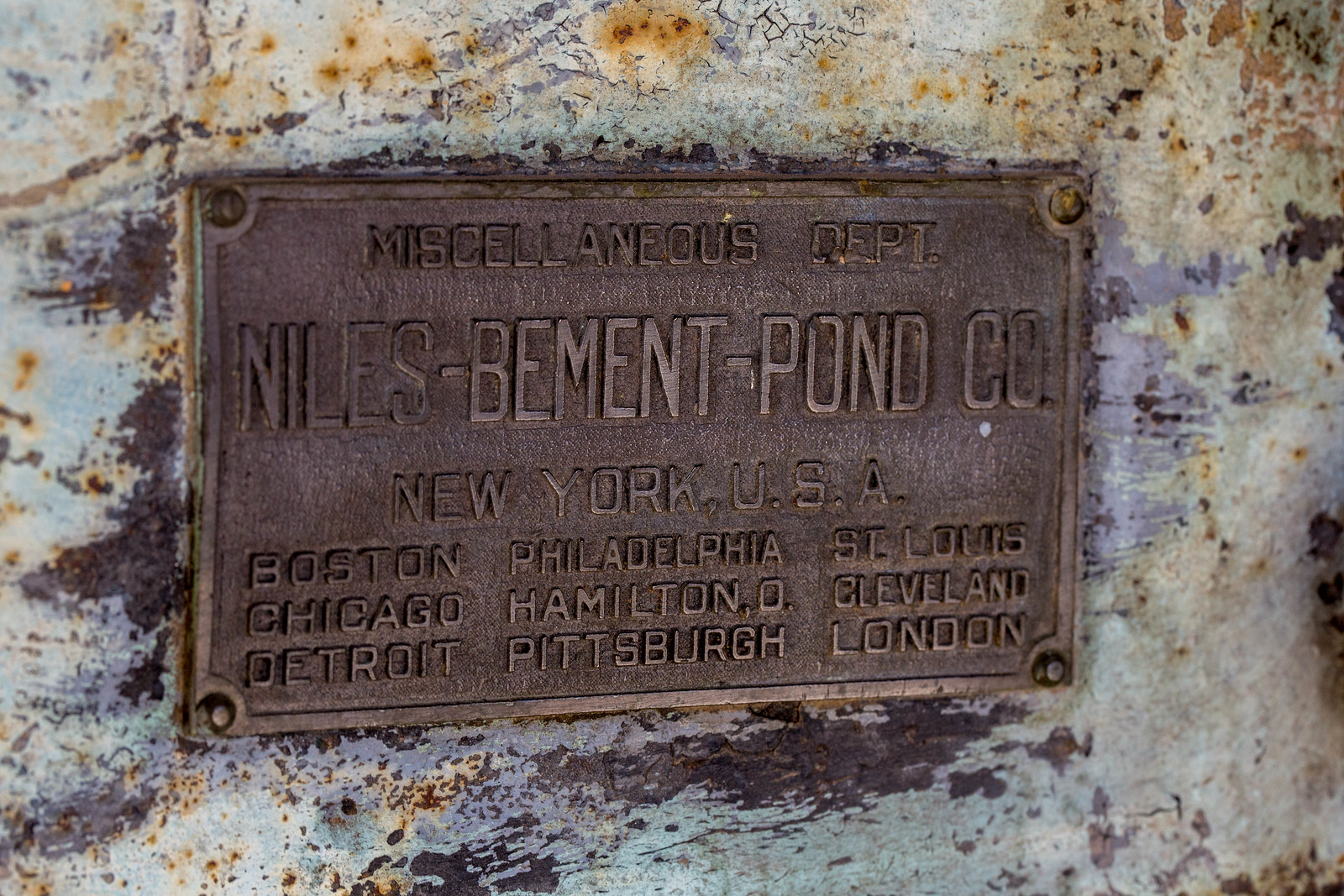This image depicts a weathered copper plaque with slightly rusted bolts at each of the four corners. The plaque belongs to the Niles-Bement-Pond Company, based out of New York, USA, under its Miscellaneous Department. It lists several other locations including Boston, Philadelphia, St. Louis, Chicago, Hamilton, Cleveland, Detroit, Pittsburgh, and London. The background appears to be an old, possibly mold-covered wall or rusted metal surface, exhibiting patches of orange and dark brown discoloration with fuzzy edges, and black spores to the left of the plaque. Despite some rusting, the plaque remains relatively intact and readable, adding a historic feel to the aged surroundings.